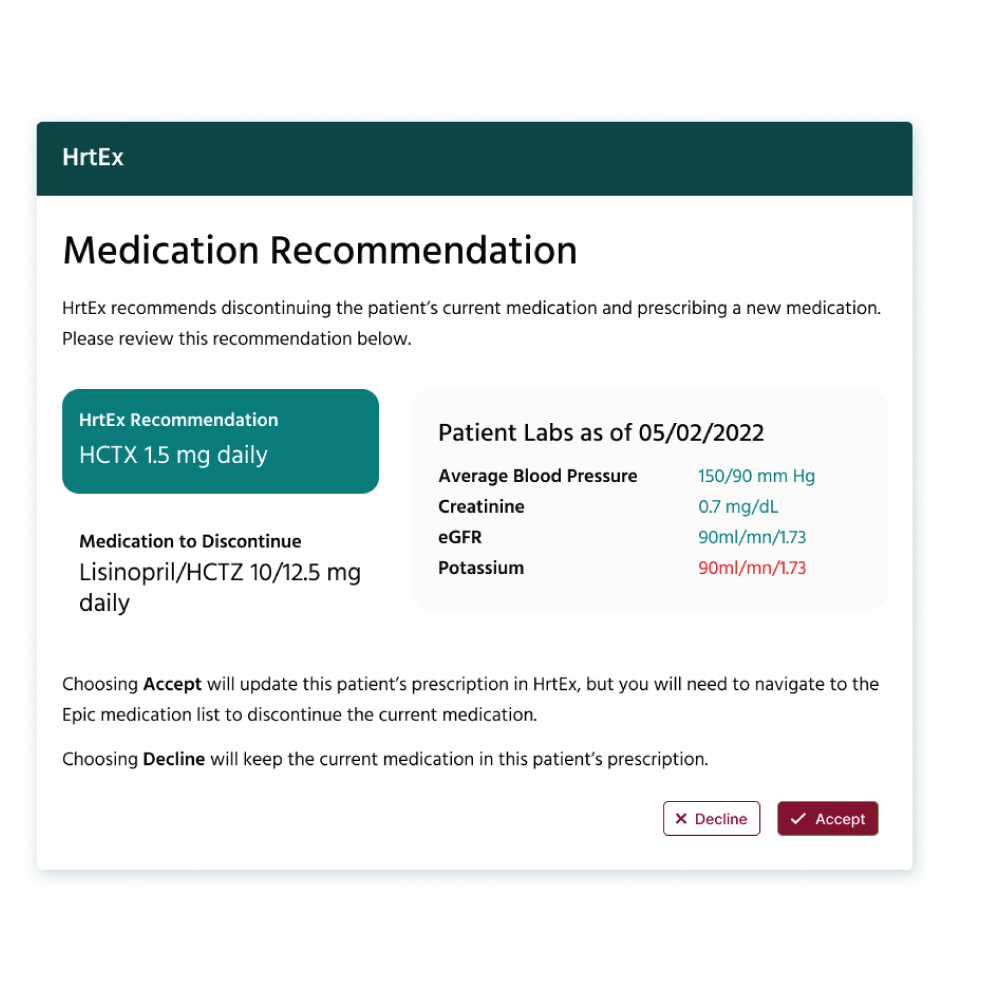The image displays a detailed medical recommendation notice from a system called Heart X. The notice is divided into several sections:

**Header:**
- **Background:** Dark green
- **Text:** Written in white, located at the top left corner, displaying "Heart X" (stylized as "HRTX").

**Main Body:**
- **Top Section:** 
  - **Background:** White
  - **Text:** Written in black, reads:
    ```
    Medication Recommendation
    Heart X recommends discontinuing the patient's current medication and prescribing a new medication. Please review this recommendation below.
    ```

**Buttons and Information:**
- **Left Side:**
  - **Button:** Dark green with white text, reading "Heart X Recommendation HCTX 1.5 milligrams daily."
  - Below the button, black text reads, "Medication to discontinue: Lisinopril HCTZ 10/12.5 milligrams daily."

- **Right Side:**
  - Text provides detailed patient data, specifically:
    ```
    Patient details as of 05-02-2022:
    Average blood pressure: 150/90 mmHg
    Creatinine: 0.7 mg
    eGFR: 90 ml/min/1.73m²
    Potassium: 90 ml
    ```
    - The numbers are color-coded: Green for all metrics except Potassium, which is in red.

**Footer:**
- **Left Side:** Instructions in black text:
    ```
    Choosing "Accept" will update this patient's prescription in Heart X, but you will need to navigate to the Epic medication list to discontinue the current medication. Choosing "Decline" will keep the current medication in the patient's prescription.
    ```

- **Right Side:** 
  - Two buttons:
    - "Accept" button: Red
    - "Decline" button: Outlined in a red border

The image overall provides a clear and comprehensive format for reviewing and acting upon a patient’s medication recommendations.